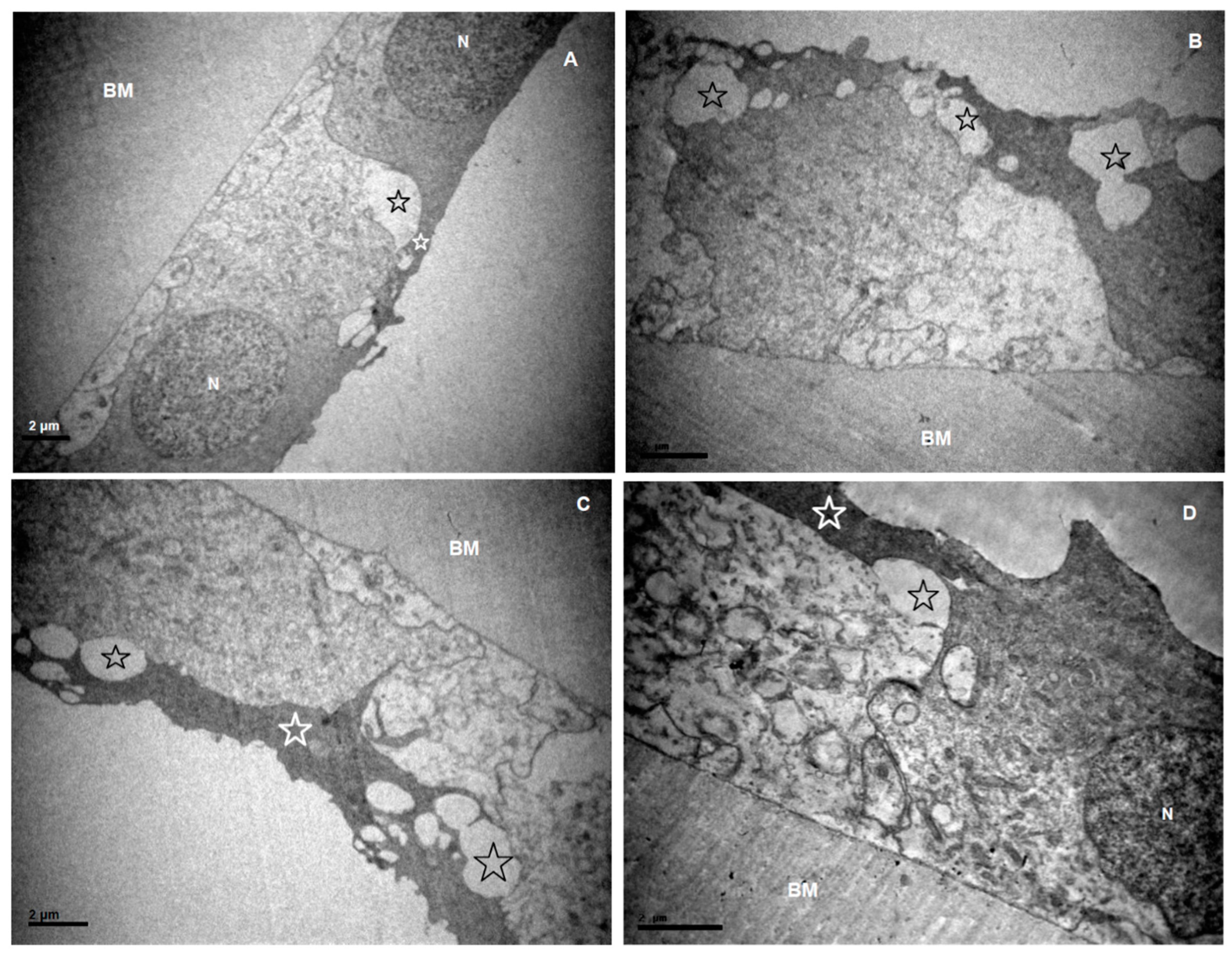The image consists of four black-and-white photographs arranged in a quadrant format, each labeled A through D starting from the top right and moving clockwise to the bottom left. Each photograph appears to be an aerial view of some deteriorated landmass or structure, characterized by shades of black, gray, and white, possibly hinting at the image's age. The photographs, taken from different angles or at different times, capture a strip-like area that shows varying degrees of decay and irregular patterns. Each photograph contains the letters "BM" positioned somewhere within the frame. There are also stars marking specific locations: one star in Image A, two stars in Image B, three stars in Image C, and two stars in Image D. Despite the differences in star counts and strip patterns, the images share a similar grayscale tone, giving them a uniform, yet enigmatic appearance.